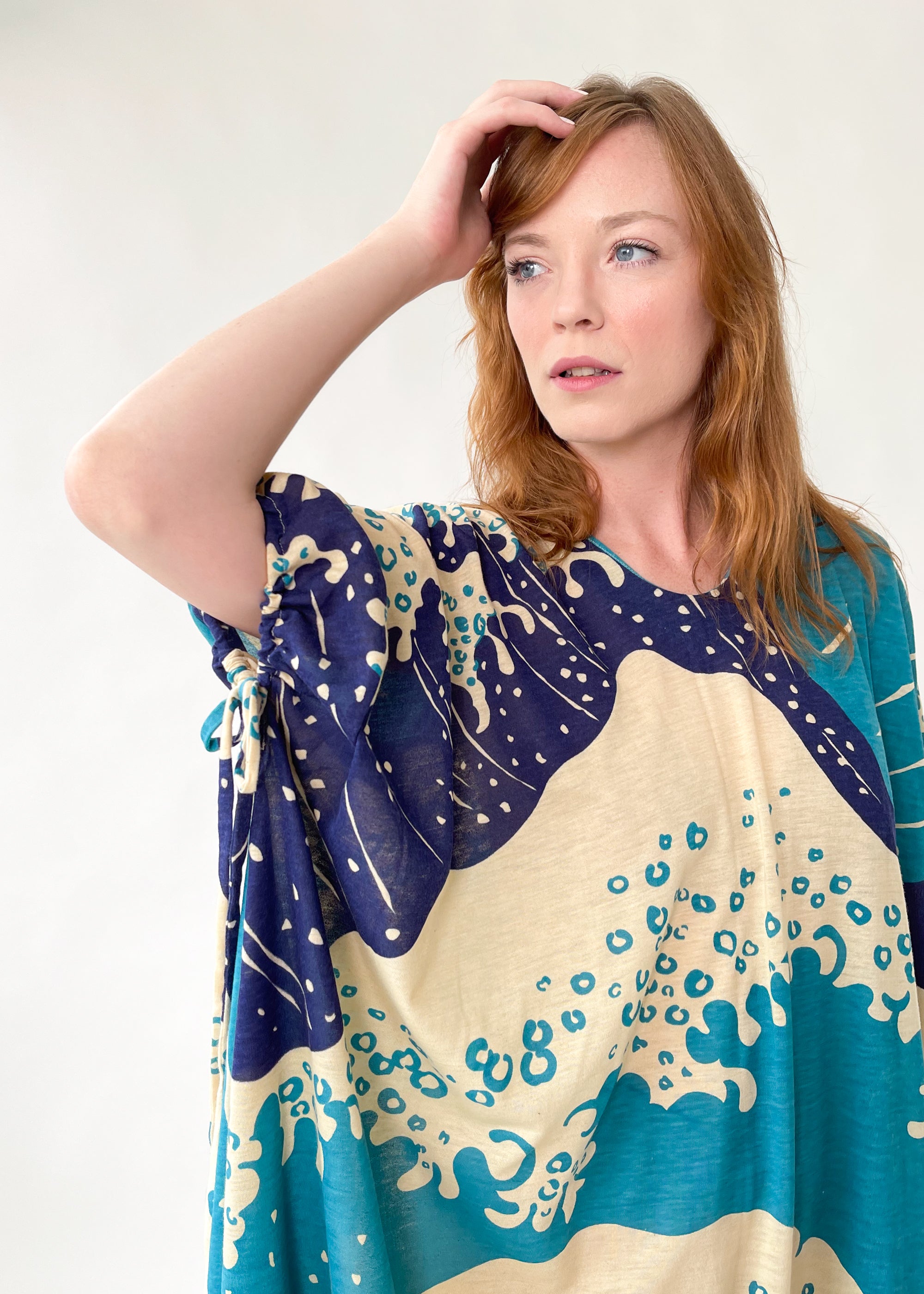The photograph is a full-color, vertical shot taken indoors under artificial light, showcasing a Caucasian young woman with striking red hair and pale complexion. Her flowing, straight hair reaches her shoulders, with slight curls towards the ends. She possesses light blue eyes, a rare combination for a redhead, and she is posing with her right arm raised to her head, fingers running through her hair, while glancing to the left.

The model is dressed in an ocean-themed caftan or poncho, which drapes elegantly over her upper body, revealing only her arms. The garment features an intricate pattern of dark blue, light blue, turquoise, and white, depicting stylized waves and seafoam bubbles, reminiscent of Polynesian or Asian art. The backdrop is a simple gray wall, keeping the focus entirely on the model and her distinctive attire.